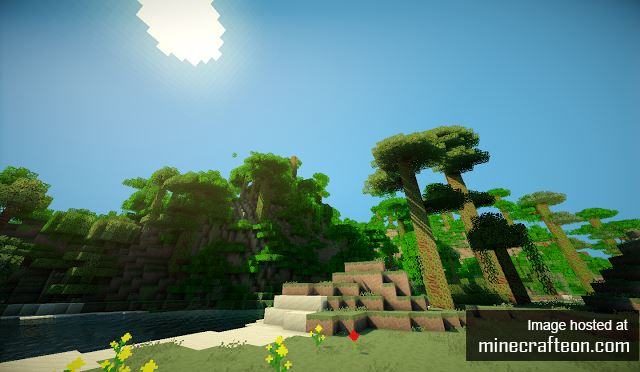This image is a screenshot from the video game Minecraft, identified by a watermark in the bottom right corner that says "image hosted at minecraftian.com." The scene is dominated by a vibrant blue sky with a distinct, blocky white sun at the top of the frame. Central to the image are several Minecraft trees of varying heights. Below these trees lies a small, blocky hill adorned with patches of grass and a few flowering bushes, featuring red and yellow flowers. On the left side of the image, there appears to be a shaded area under additional trees, possibly hinting at a stream or body of water between them. The entire scene is rendered in the characteristic pixelated style of Minecraft, with all elements—trees, flowers, sun, and hills—displaying the game's iconic blocky design.